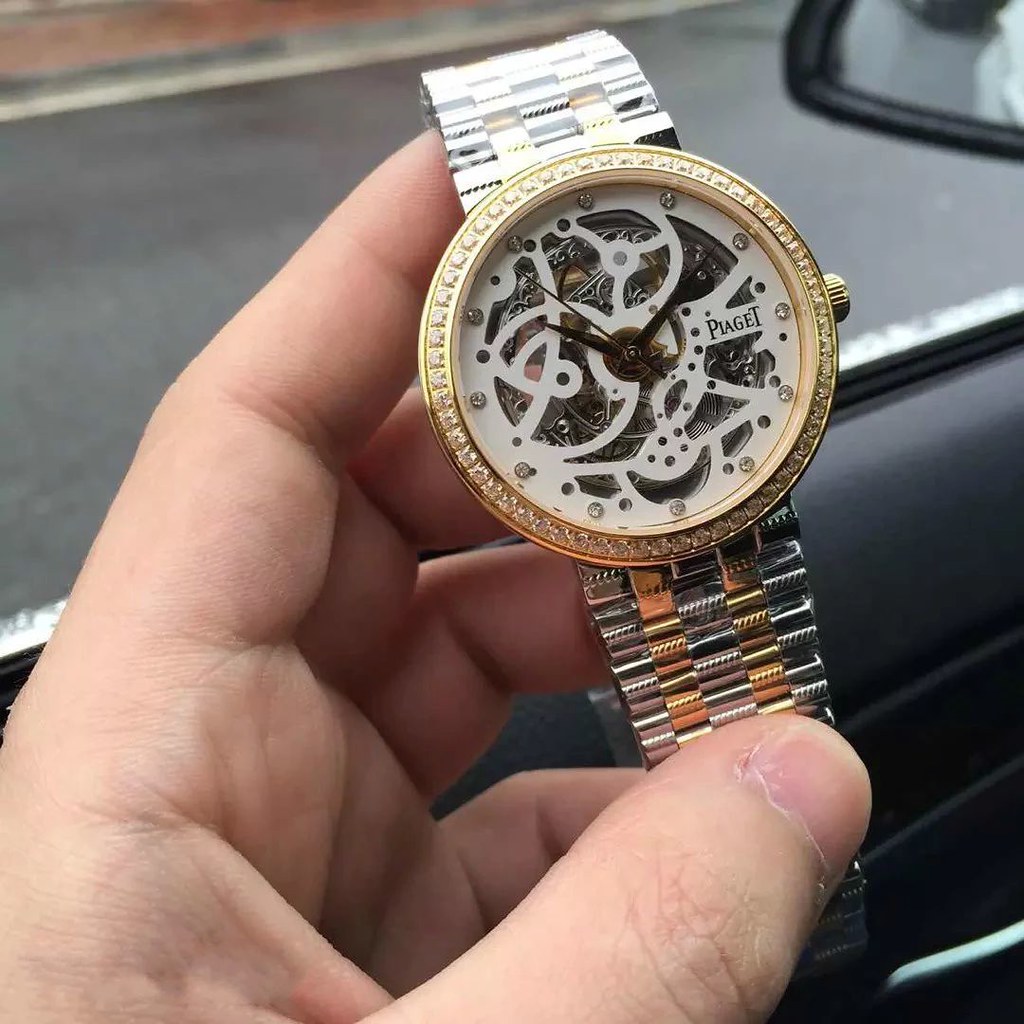In this close-up shot, a Piaget watch is elegantly displayed by a man as he exits a vehicle. The man holds the watch delicately, with the top of the watch band resting on his index finger, his middle finger supporting the back of the watch, his ring finger touching the bottom inside of the band, and his thumb grasping the band from the outside. The background reveals a rainy scene, evidenced by the wet sheen on the road visible in the upper part of the photo, along with glimpses of the driver's side door at the bottom and a partial view of the rear-view mirror in the top right corner.

The Piaget watch is a stunning blend of gold and silver, with a silver band accented by gold links running through the center. The watch face is bordered in gold and adorned with tiny diamonds. Inside the gold bezel, the white watch face also glistens with diamonds marking the hours. The intricate, mechanical design of the watch face allows a view of the inner workings, showcasing cog wheels and other components. The brown watch hands stand out against the watch face, indicating the time at 10:10.